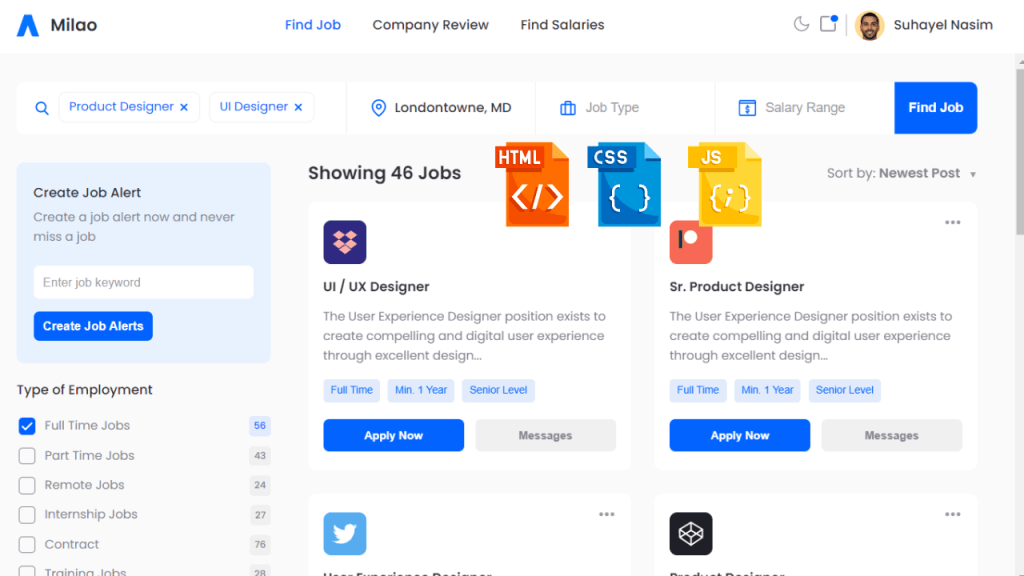Screenshot of a job search website featuring the name "M-I-L-A-O" at the top with an icon next to it. The page includes sections for finding jobs, company reviews, and salary information. On the right, there's an avatar indicating the user's profile. The interface shows an option to create job alerts, with a list of 46 job opportunities in fields such as UX/UI Design, Senior Product Design, HTML, CSS, and JavaScript. These jobs are sorted by the newest postings. Each job listing includes a brief description and options to apply immediately through a prominent blue "Apply Now" button, or to send messages via a gray "Messages" button. The background of the page is light blue with sections to enter job keywords. There are filters for different job types like full-time, part-time, remote, internship, and contract positions, with the full-time filter highlighted by a blue box and white checkmark.